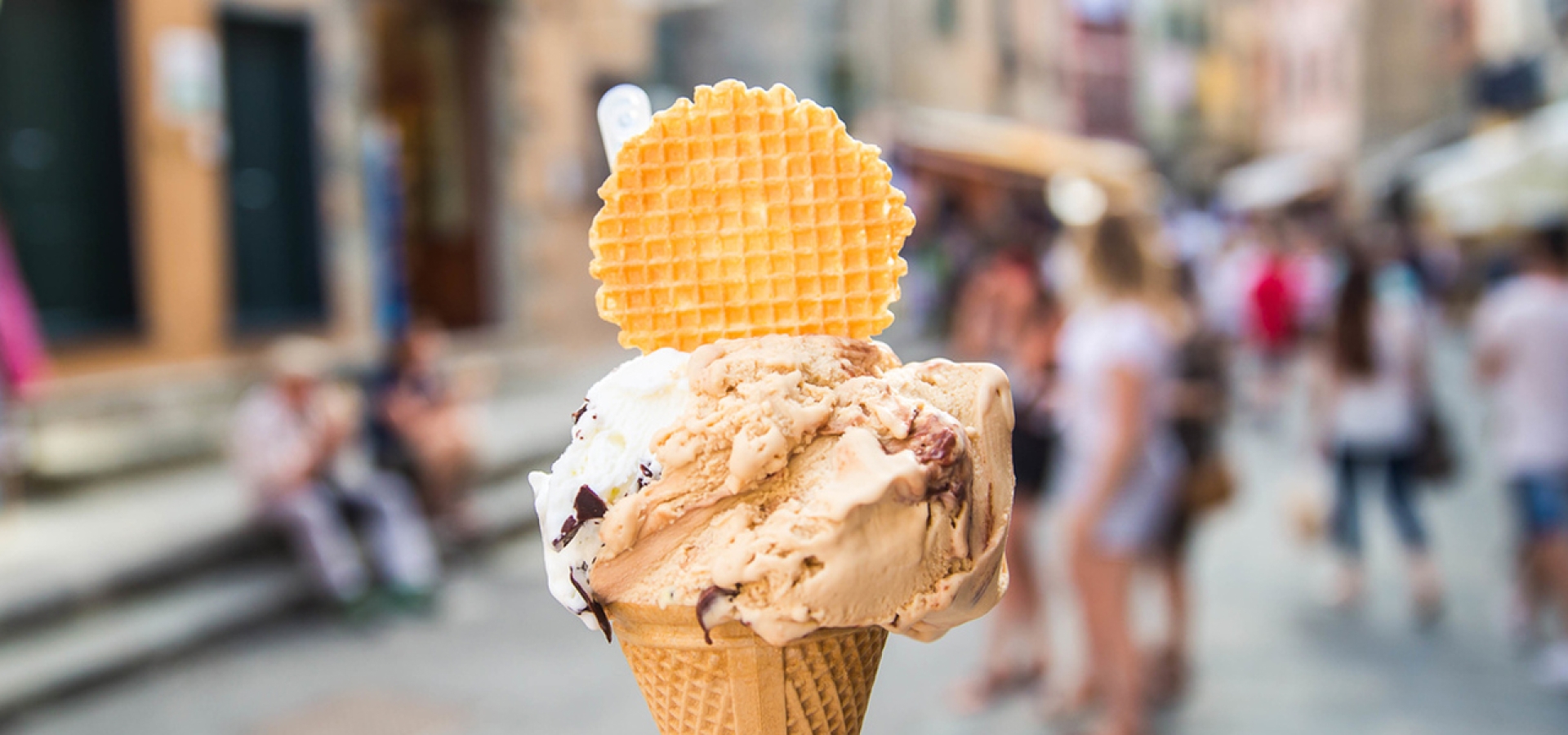This rectangular photograph, taken in a portrait orientation, features a delectable ice cream cone prominently in the foreground, with the background artistically blurred. The visible portion of the cone starts from its midsection upward, showcasing its tan-colored waffle exterior adorned with a latticework pattern. Perched on top is a generous serving of two distinctive ice cream flavors: one side is creamy white with black chocolate bits, likely vanilla, while the other is a light tan hue with dark brown nutty chunks, possibly coffee or caramel. Adding a whimsical touch, a round waffle cookie resembling a miniature Eggo waffle is inserted into the top of the ice cream, slightly obscuring a spoon's tab behind it. Faintly discernible in the blurred background are colorful buildings and various people, including a couple sitting on steps, perhaps savoring their own frosty treats, adding to the lively ambiance of the setting.